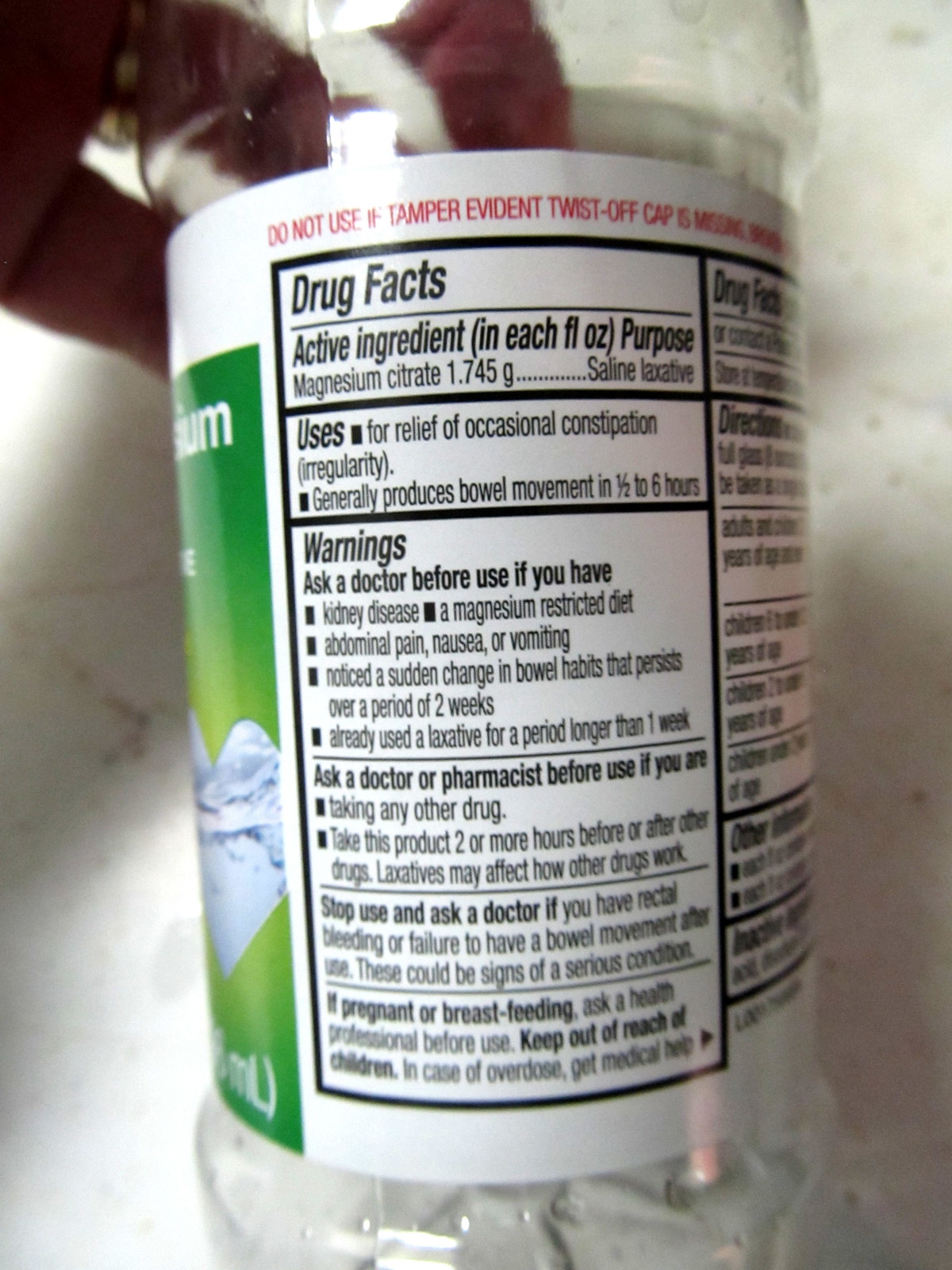This detailed close-up photograph captures the side of a clear plastic supplement bottle that appears to be empty. The bottle is transparent, allowing a glimpse of dark-skinned fingers inside the top, as if someone is trying to retrieve the remaining contents. The bottle features a detailed drug facts label prominently displayed on the side. The label indicates that the active ingredient in the supplement is magnesium citrate, which is classified as a saline laxative.

The text specifies its purpose as providing relief from occasional constipation and irregularity, with the expected action window being between half an hour to six hours. The label also includes crucial warnings and usage instructions, such as advising pregnant or breastfeeding individuals to consult a health professional before using the product. It emphasizes keeping the supplement out of reach of children and details the necessary actions in case of an overdose.

The scene is set on a white linoleum counter adorned with gold veins, providing a contrasting background to the see-through bottle and its detailed label.